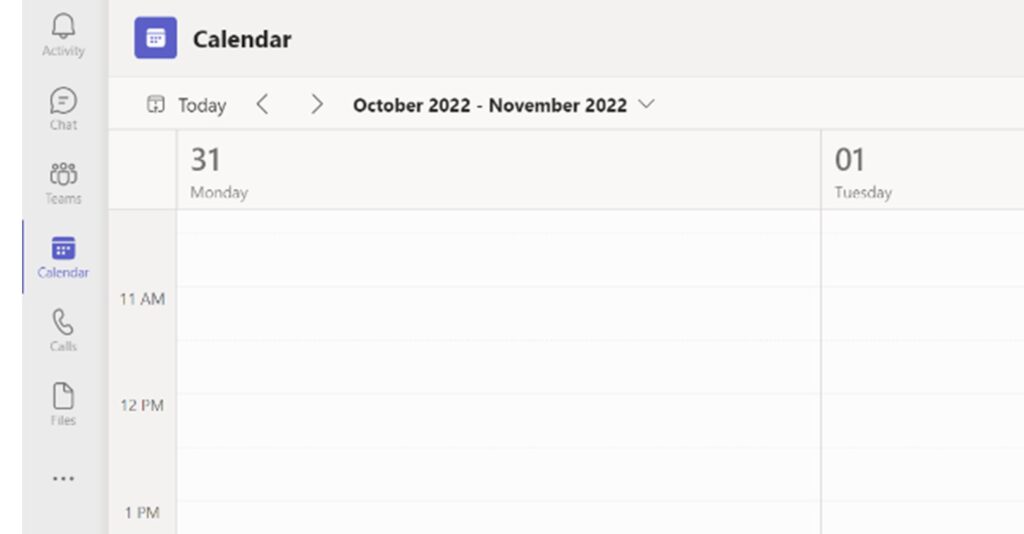The image depicts a minimalistic screenshot taken from an unspecified calendar application. The interface sports a mix of gray, off-white, and white tones. On the left-hand side, there is a vertical column featuring a series of gray icons and labels:

- At the top, a notification bell icon labeled "Activity".
- Below it, a chat bubble icon labeled "Chat".
- A figure of three people labeled "Teams".
- A calendar icon labeled "Calendar", highlighted with a purple line on its left side.
- A receiver icon labeled "Calls".
- A piece of paper with a dog-ear labeled "Files".

At the bottom of this column are three gray horizontal dots.

In the top-left corner of the main section, a purple square icon with a white calendar at its center is visible. To its right, "Calendar" is written in bold black text. Below this header text:

- On the left, the word "Today".
- Next to "Today" are left and right arrow icons.
- Following the arrows, the date range "October 2022 to November 2022" is displayed in bold, accompanied by a down arrow.

Next, a large gray banner displays "31 Monday" in gray lettering, and to its far right, the columns start anew with "01 Tuesday".

Furthermore, on the left-hand side, there are time labels marking "11 a.m.", "12 p.m.", and "1 p.m." 

Overall, the design is quite sparse, focusing on a clean and organized layout for easy navigation within the calendar application.